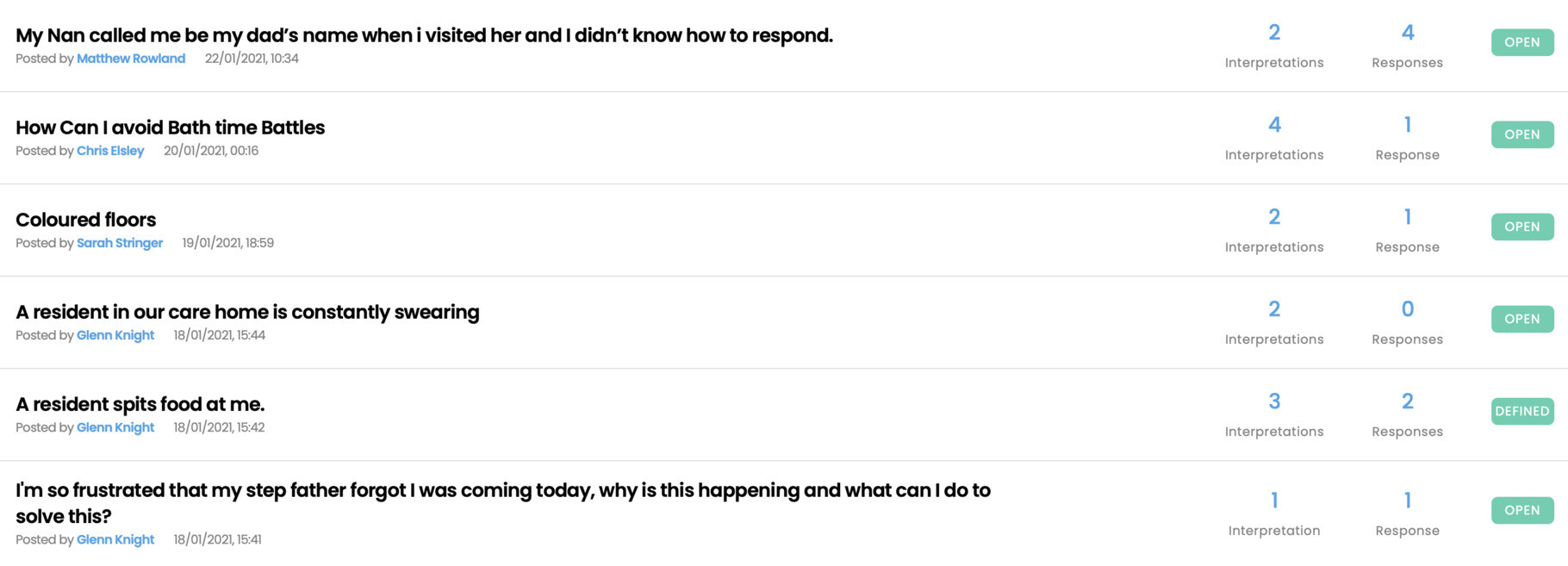The image features a light gray, almost white background and appears small and blurry. In the middle section, there are four notable columns. The leftmost column contains a series of brief text entries, each followed by a name and date, likely indicating the person who posted and the time of posting.

Starting from the top, the first entry reads: "My Nan called me by my Dad's name when I visited her, and I didn't know how to respond," accompanied by the poster's name and a timestamp, followed by a horizontal line. Below this, another entry asks: "How can I avoid bath time battles?" posted by an individual named Chris, and is also accompanied by a date and time, followed by another horizontal line. Further down, an entry mentions: "A resident in our care home is constantly swearing," with the poster's name and timestamp below it. Lastly, an entry reads: "A resident spits food at me," followed again by the poster's details and posting time. 

At the bottom of the left column, one more entry states: "I'm so frustrated my stepfather forgot I was coming today; why is this happening, and what can I do to solve this?" Each post is demarcated by a horizontal line separating it from the next.

On the right side of the image, there are three columns, each aligned vertically and containing numbers. Each of these columns features a green button, likely signifying an action such as approval or selection, corresponding to the respective entries.

This descriptive arrange captures the essence and details of the original image while providing clarity and structure.